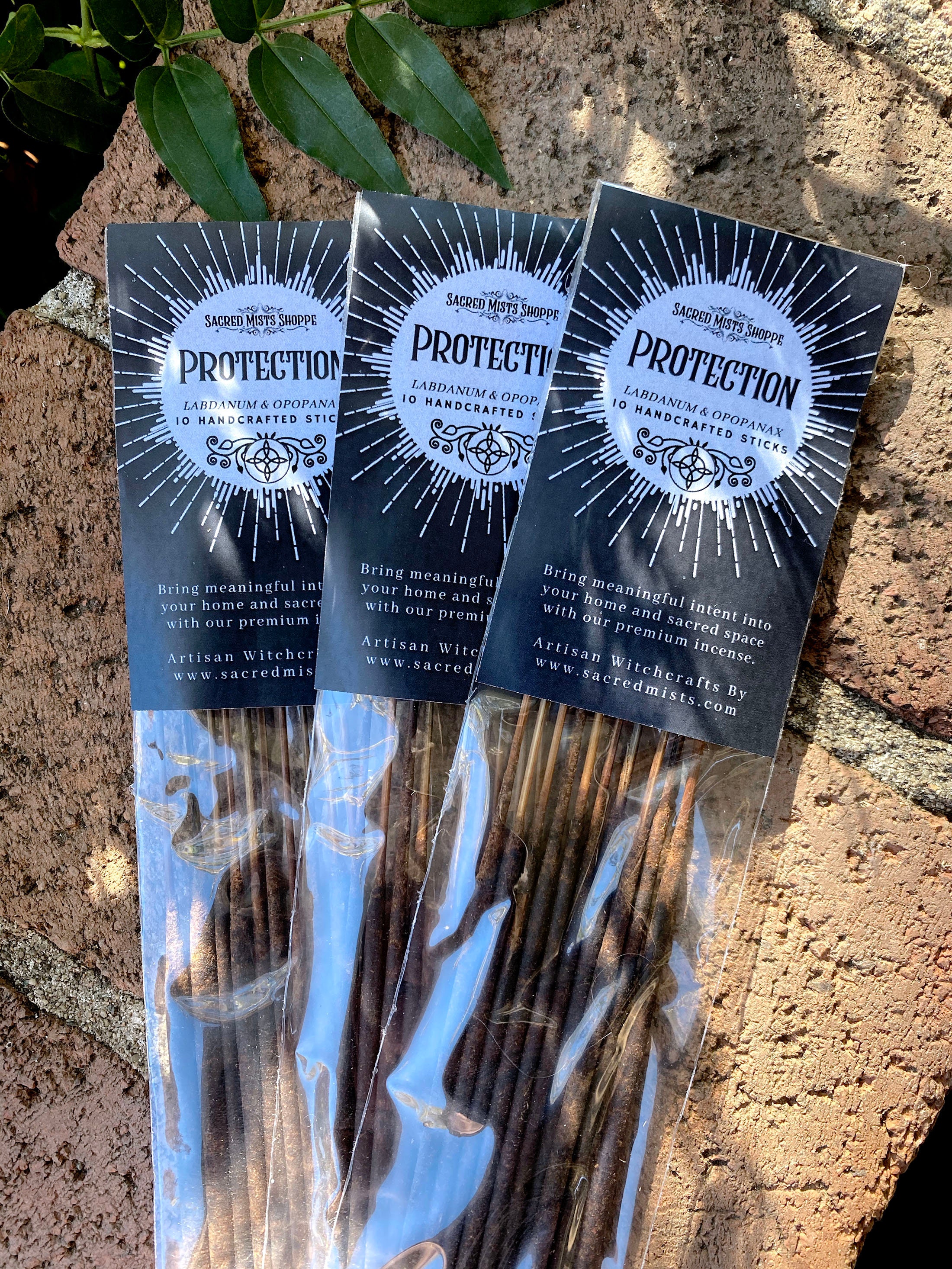The photograph captures an outdoor scene featuring three identical packages of handcrafted incense sticks from Sacred Mists Shop, artfully displayed atop light worn-out terracotta bricks with gray grout. The three narrow, rectangular packages are arranged in a slightly fanned-out manner, akin to spreading a deck of cards. In the upper left-hand corner, three green leaves add a touch of natural greenery to the composition.

Each package sports a striking black and white label at the top, showcasing a decorative swirl pattern within several concentric circles, all enclosed within a blue sunburst design. The label reads: "Sacred Mists Shop, Protection, Labdanum, 10 handcrafted sticks." Below this, white lettering invites the viewer to "Bring meaningful intent into your home and sacred space with our premium incense. Artisan Witchcrafts by www.sacredmists.com."

The lower half of each package is made of clear cellophane, revealing the neatly arranged brown incense sticks inside. The combination of the detailed label, the clear plastic revealing the product, and the natural outdoor setting creates a visually appealing and serene presentation.